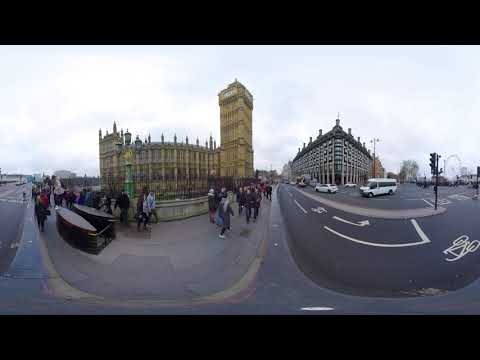The image depicts a scene captured with a fisheye lens, distorting the elements into a convex view. To the left, a three-story, yellowish-tan ornate building stands with a prominent tower on its right side, featuring a clock at the top. Surrounding this building, a bustling crowd navigates the curved sidewalk that encircles it, exaggerated by the fisheye effect. On the street nearby, unidentified black objects resembling canoes or kayaks can be seen. The building on the right side of the frame is grey and equally ornate, topped with a cross and standing several stories tall. A white van and a white car are parked in front of it, amidst other vehicles in the distance. A street light with a crossing signal stands near the bottom right corner where an arrow and bicycle markings are visible on the curved pavement. The sky above is softly clouded, signaling daytime.